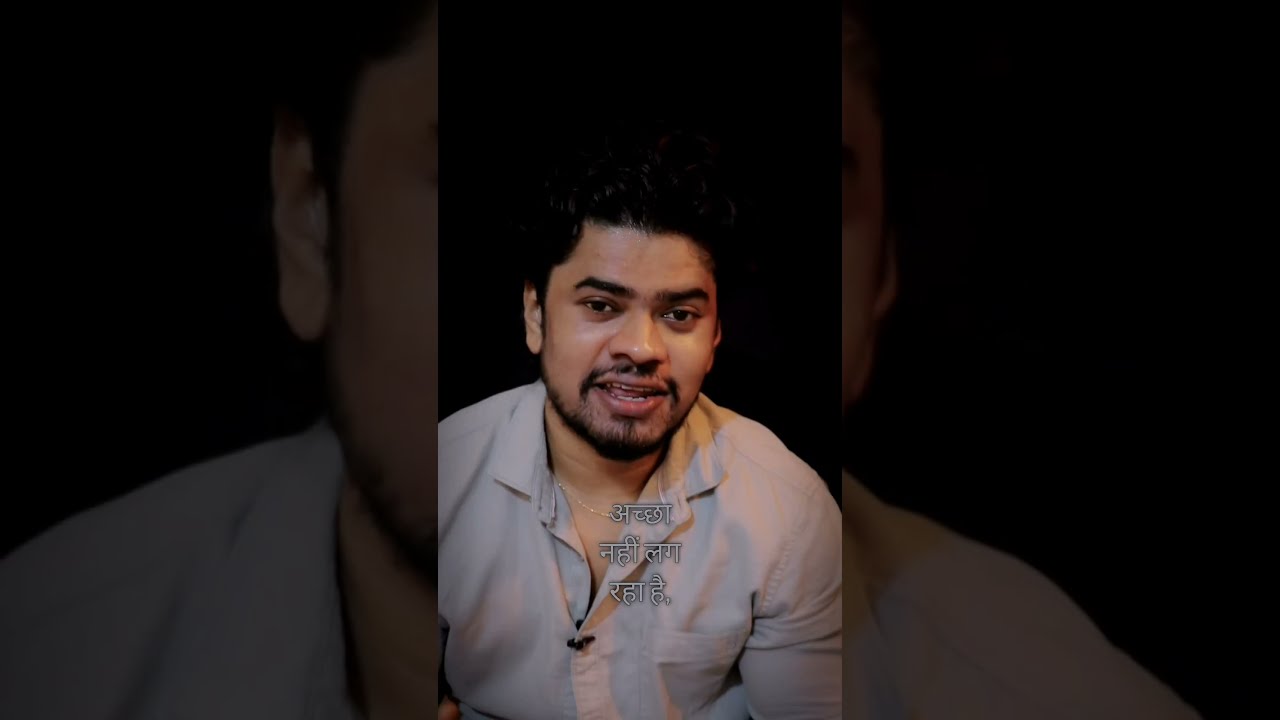This image is a composite portrait of a man, divided into three segments with the outer segments being zoomed-in portions of the left and right sides of the central image. The man, possibly Hispanic or Indian, is shown from just above the elbow up, with a muscular build and his arms pressed to his sides. He faces the camera with his mouth partially open, as if speaking, and is adorned with a black mustache, beard, and short black hair. His attire consists of a tan or cream-colored, unbuttoned collared shirt, revealing a small golden chain around his neck and a microphone attached to his chest. The entire background is black, making the subject stand out prominently. Additionally, there is white text in what appears to be Arabic script overlaying his image. The man's detailed facial features include black eyebrows, dark eyes, and a wide nose, with his gaze directed slightly off to the side.